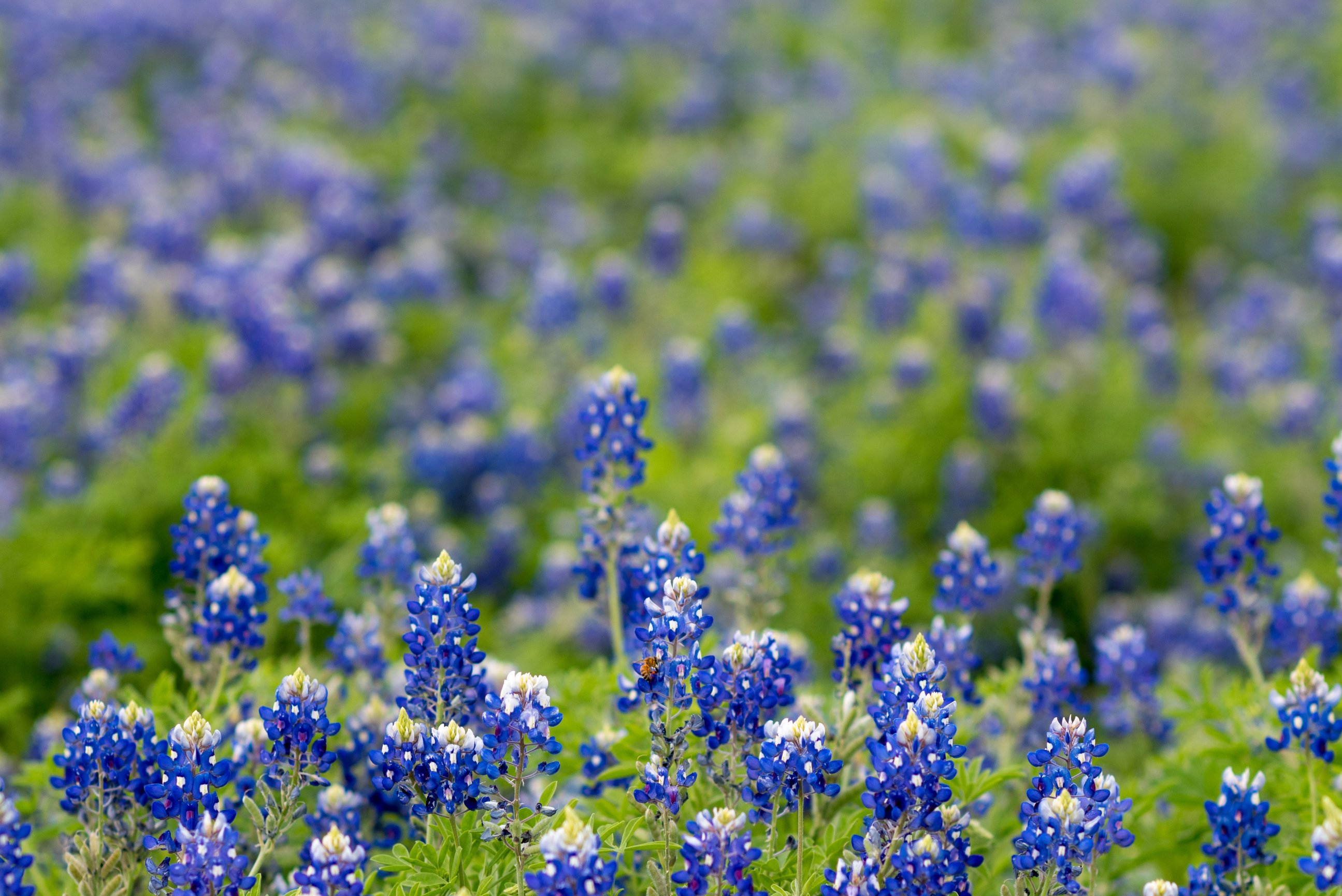The image captures a picturesque field of blooming flowers extending into the distance. The foreground is sharply focused, showcasing an array of flower stalks adorned with brilliant blue-purple petals. Each flower exhibits clusters of lush, compact petals with tiny white and yellow centers. Some flower stalks culminate in white bulbs at their tips. The vibrant blooms rise gracefully above a bed of green foliage, which appears almost grass-like. The background, occupying the top two-thirds of the image, is beautifully blurred, hinting at the vastness of the field stretching far into the distance on a bright, sunny day. The overall scene is a harmonious blend of blue, white, and green tones, exuding a sense of endless natural beauty.